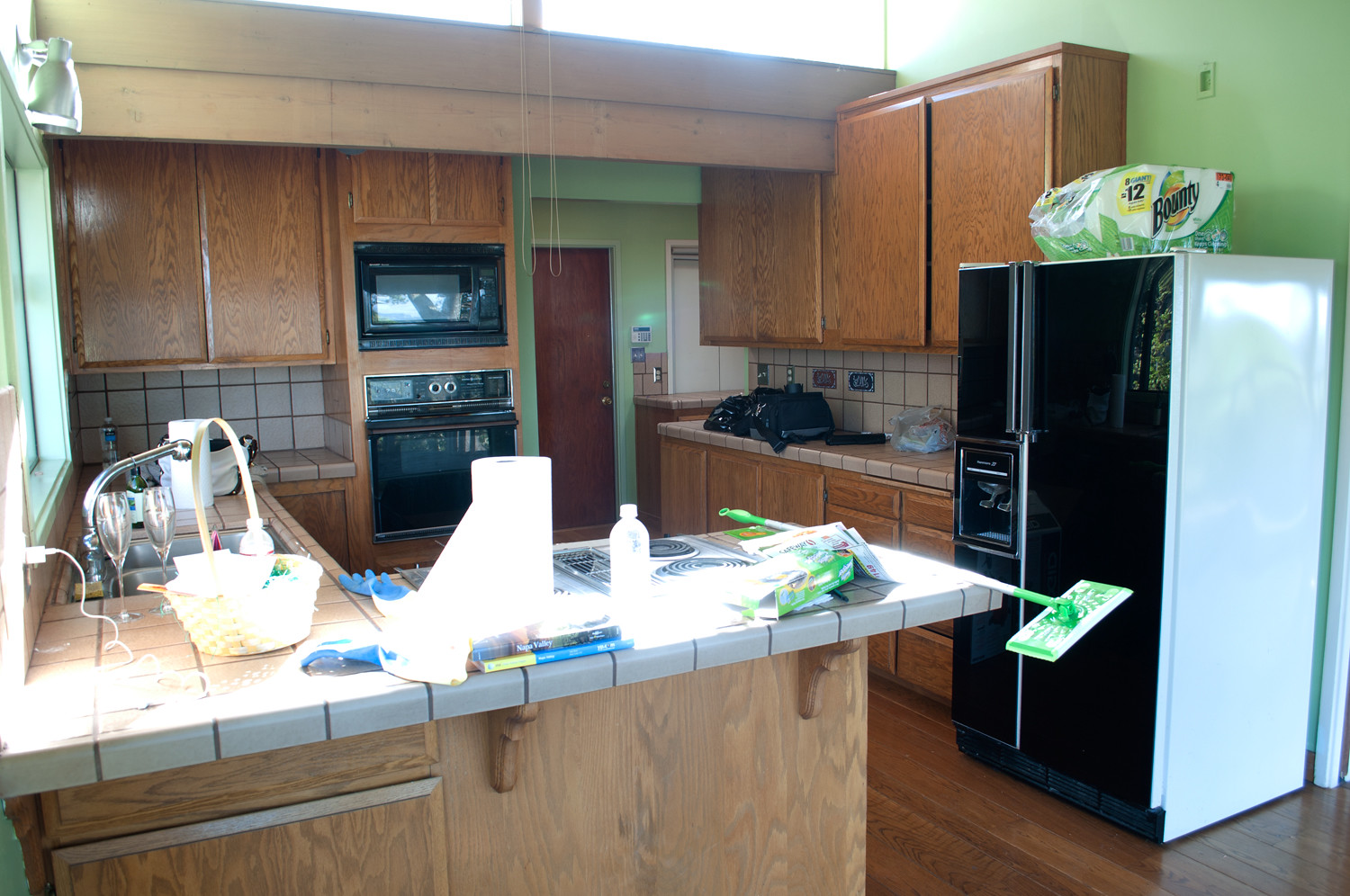The photograph captures a busy kitchen, evidently in the midst of a cleaning session. The back wall features a section of counter space adorned with small, off-white tiled backsplash and countertop. To the far left, there's a set of brown cabinets without handles. Adjacent to these cabinets sits a black microwave, itself topped by two small square doors and underlain by a matching black oven. The scene extends to the right, revealing a hallway with green walls and a large wooden door.

Directly forward, the kitchen boasts another countertop area, also with off-white tiled surface, accompanied by three overhead cabinets and several cabinets and drawers below. Scattered on this countertop are some black items, likely trash bags, indicating the cleaning in progress. To the far right, a refrigerator with a black front and white sides stands prominently.

In the top left corner of the image, a bar countertop comes into view, hosting a roll of paper towels and a package that appears to contain mop pads. A mop dangles off this counter, with its head hanging towards the right. The entire kitchen is tied together by dark wood flooring, adding warmth to the space amidst the cleaning activity.